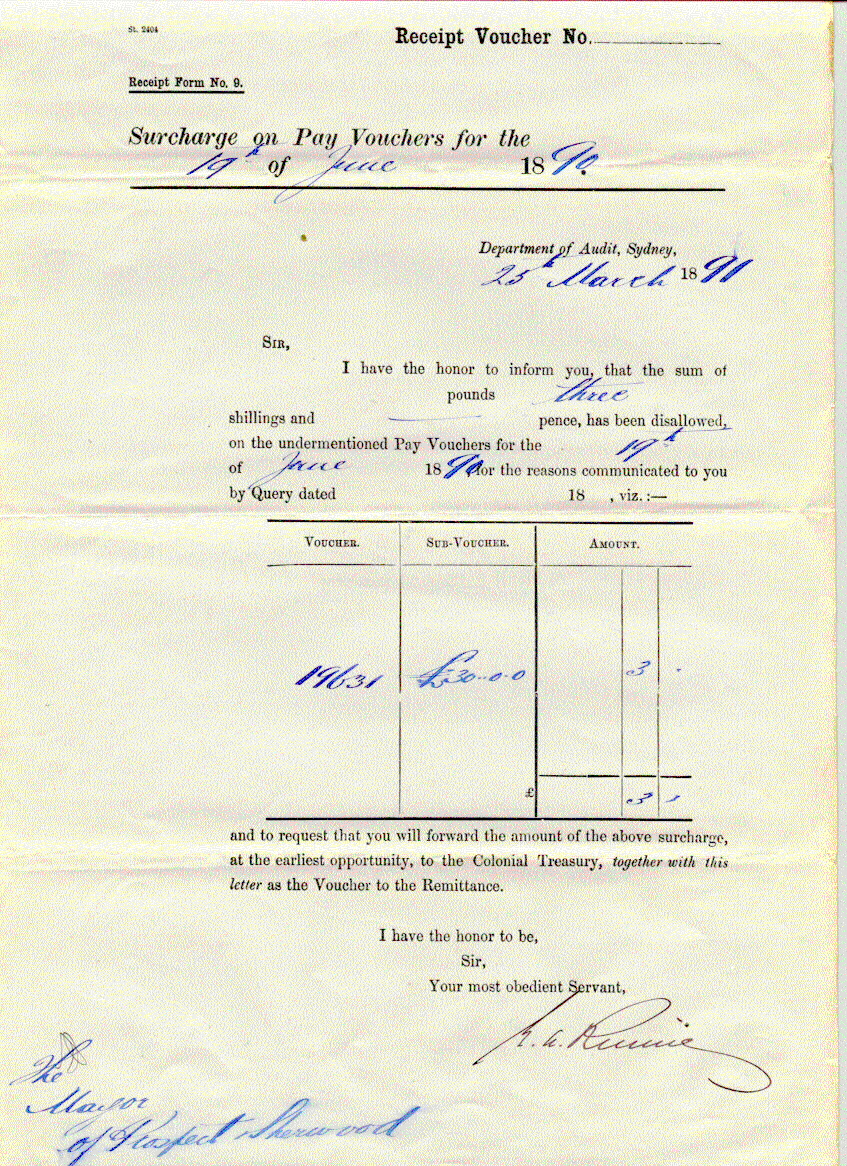The image displays a yellowed and aged receipt voucher, prominently titled "Voucher Receipt" at the top. The document bears the "Voucher Number" and "Receipt Form No. 9." It details a "surcharge on pay vouchers for the 19th of June, 1890," and specifies correspondence from the "Department of Audit, Sydney" dated the 25th of March, 1891. It includes formal text beginning with "Dear Sir, I have the honor to inform you that the sum of three pounds, shillings, and [blank] pence has been disallowed on the undermentioned pay vouchers for June, 1890." The document ends with the salutation, "I have the honor to be, Sir, your most obedient servant," followed by an illegible signature in black ink. Blue ink markings can be observed in certain sections of the paper.